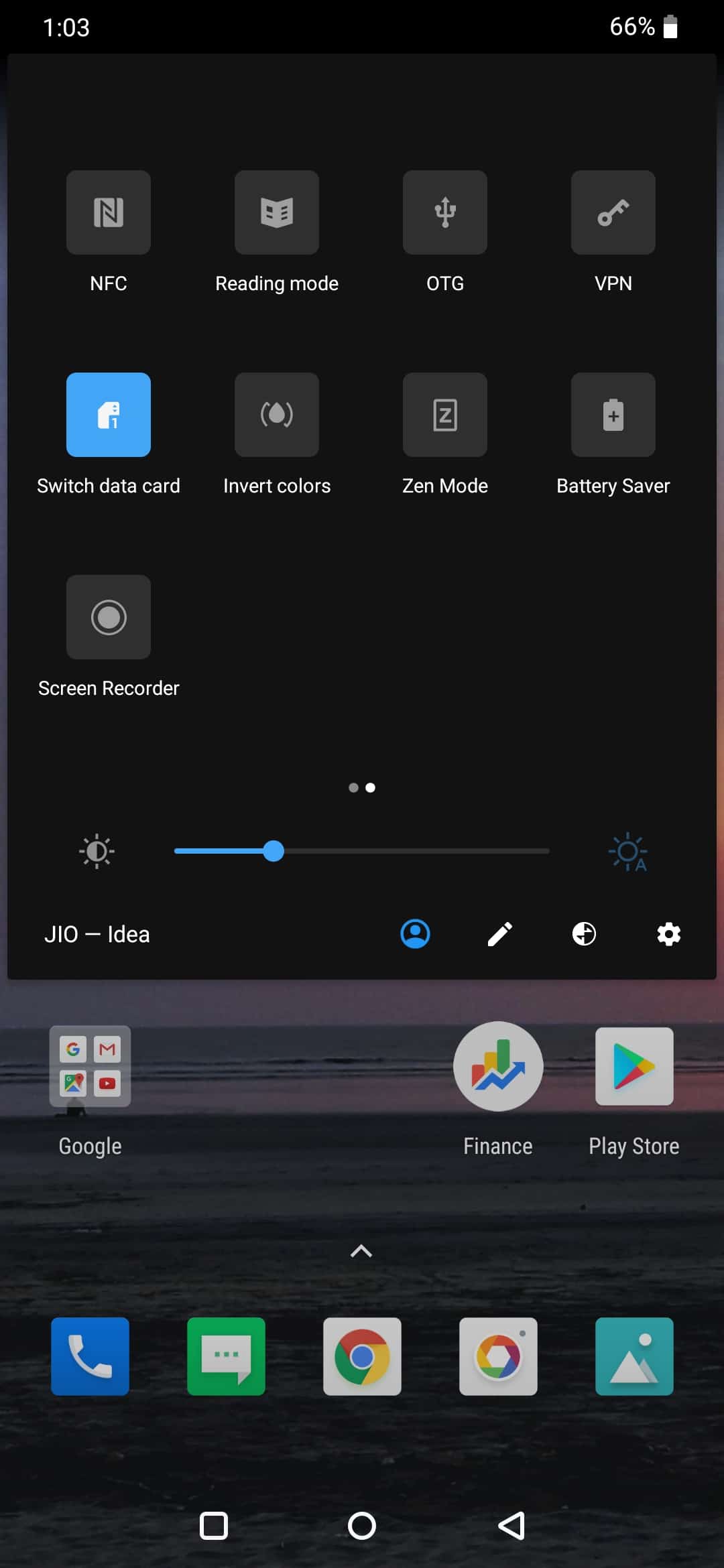This screenshot captures a detailed view of a smartphone's Quick Settings menu and home screen elements. The top row of icons showcases various functionalities: NFC (Near Field Communication), Reading Mode, OTG (On-The-Go), and VPN (Virtual Private Network). The second row displays additional options: Switch Data Card (highlighted in blue to indicate it is selected), Invert Colors, Zen Mode, Battery Saver, and Screen Recorder.

Directly below these icons is the brightness adjustment bar, which is almost slid to the left side, suggesting dim lighting. Under this bar, the text 'JIO' and '- Idea' signifies the active and inactive SIM cards, respectively. 

Further down, a small profile icon, a pencil icon (likely for editing), a circular icon, and a settings gear icon can be seen, indicating various user profiles and settings options.

At the bottom of the screen, three app icons are visible: a Google folder, a finance-related application, and the Play Store. The icons reflect the user's commonly used apps and provide quick access to essential services.